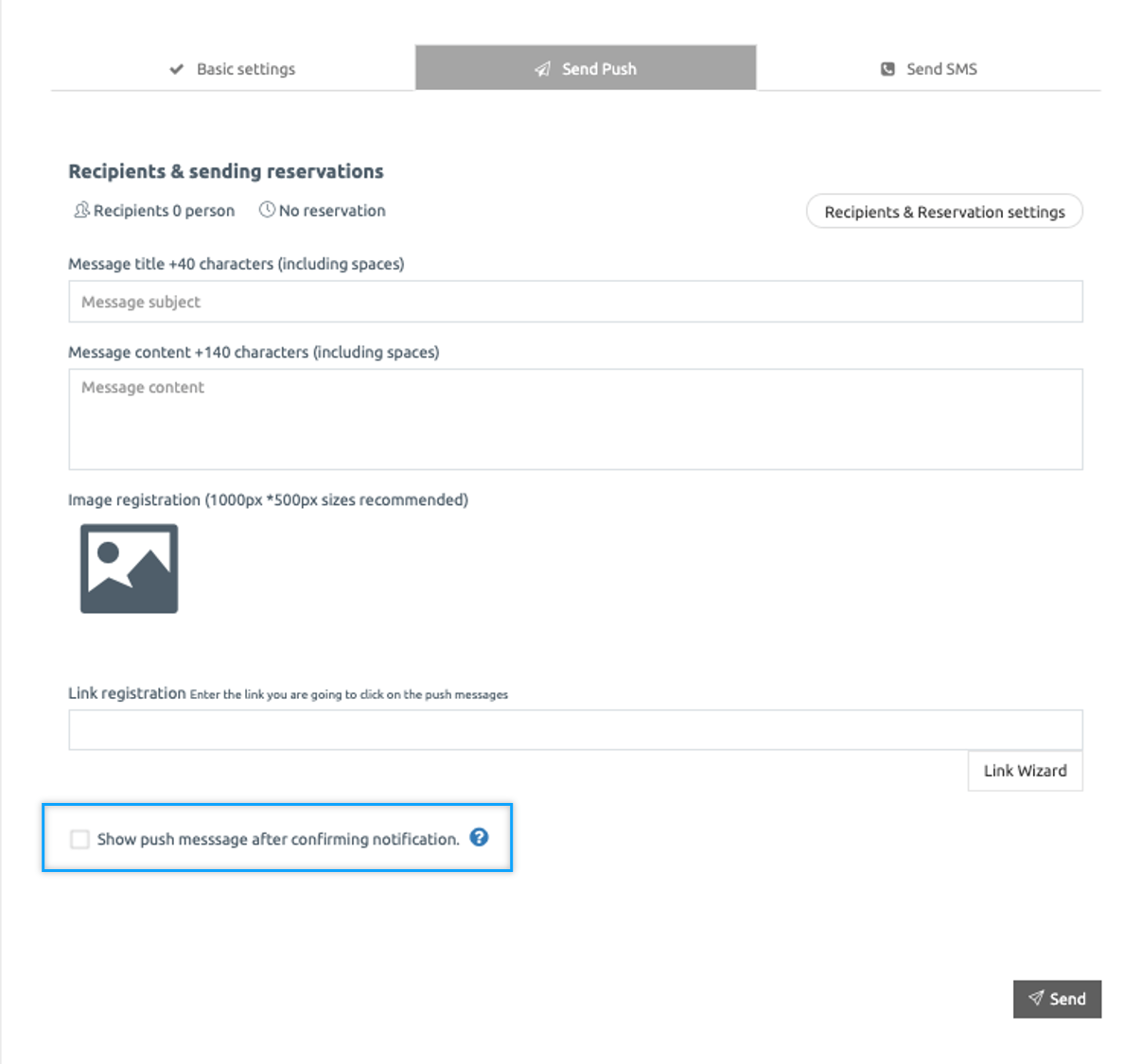The image depicts an interface commonly used for managing and sending communication messages to recipients, such as through emails or push notifications. 

In the top left corner, there is a gray checkmark icon accompanied by gray text that reads "Basic Settings." To its right, within a gray rectangular background, is the option "Send Push" followed by an airplane-like icon, indicating the ability to send push notifications. Adjacent to this, there's a gray box housing a white telephone icon, labeled "Send SMS," signifying an option to send SMS messages.

Beneath these options, there is a section labeled "Recipients and Sending Reservations." This area displays "Recipients: 0" and "Reservations: No Reservation," with a clock icon next to the reservation status, indicating the current reservation details. 

To the right, in a circular-like rectangle, there are settings for "Recipients and Reservation Settings." Below this section, there is a field labeled "Message Title," which allows for up to 40 characters, including spaces. Within this long rectangular box, "Message Subject" can be entered.

Further down, another field labeled "Message Content" is provided, allowing up to 140 characters, including spaces. This repeats with a secondary field also labeled "Message Content."

Underneath the message content fields, there is an area titled "Image Registration," which recommends an image size of 1,000 px by 500 px. A dark gray square is depicted here, featuring an icon of a mountain and sun, symbolizing where the image would be displayed.

Below, the "Link Registration" section instructs the user to "Enter the link you are going to click on the push messages." This section features a long, empty rectangular box for entering the link, with a "Link Wizard" button housed in a small rectangle to the right.

Near the bottom right, there is a white checkbox accompanied by the instruction, "Show push message after confirming notification," with a question mark in a blue circle next to it for further information. Finally, to the right of this checkbox is a gray "Send" button with white text, ready to be used for dispatching the configured message.